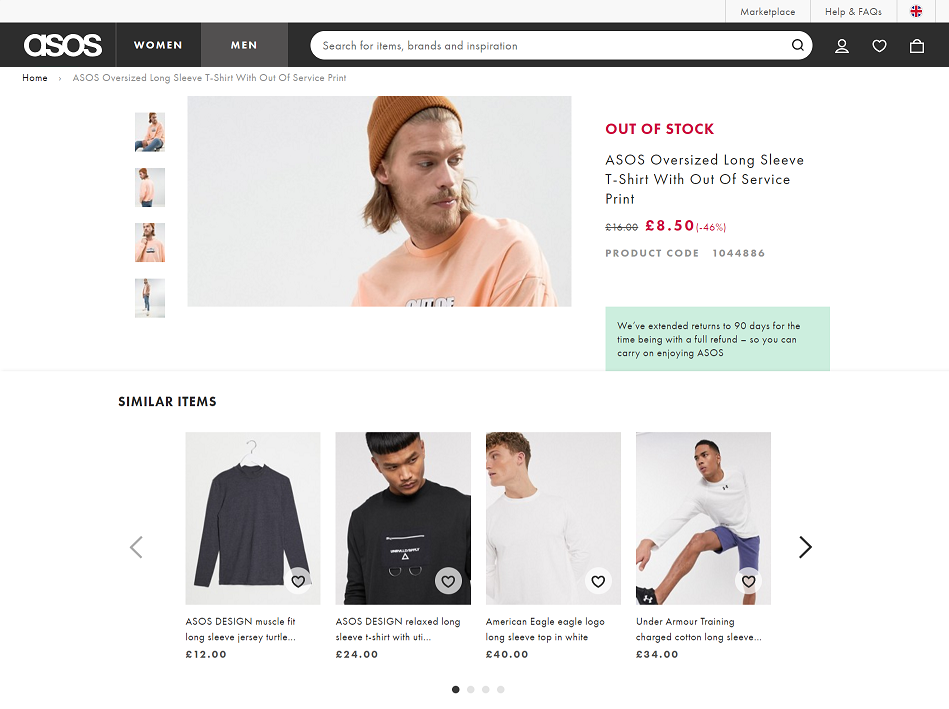**ASOS Website Banner Description**

The ASOS website features a charcoal-colored banner prominently displaying the brand's name, "ASOS," in all caps. Above this banner, there is a light gray strip that includes links to "Marketplace Help" and "FAQs" on the left. On the right side of the strip, a small circle hosts a portion of the British Union Jack, highlighting the brand's UK origins.

Across the banner, the navigation options include "Women" and "Men," with the "Men" option currently selected. A search bar spans the center, inviting users to "Search for items, brands, and inspiration." User account options are available via a guest icon that opens account personalization settings.

Below the navigation banner, the focus is on an "ASOS Oversized Long-Sleeve T-Shirt without a Service Print." This item is currently out of stock, indicated in a pinkish-red label. Originally priced at £16.99, the shirt is now offered at a discounted price of £8.50, reflecting a 46% reduction. Despite the discount, the item remains unavailable.

To the left of the product details, several images of the t-shirt are displayed, with a larger central image featuring a model wearing the shirt. An announcement beneath the product highlights that ASOS has extended its return policy to 90 days, offering a full refund to ensure customer satisfaction.

Below the main product listing, a selection of "Similar Items" is showcased. This section includes various brands such as American Eagle, Under Armour, and ASOS Design. However, the items displayed differ significantly in style, with the primary commonality being long sleeves. Four alternative options are presented, though they do not closely resemble the featured t-shirt.